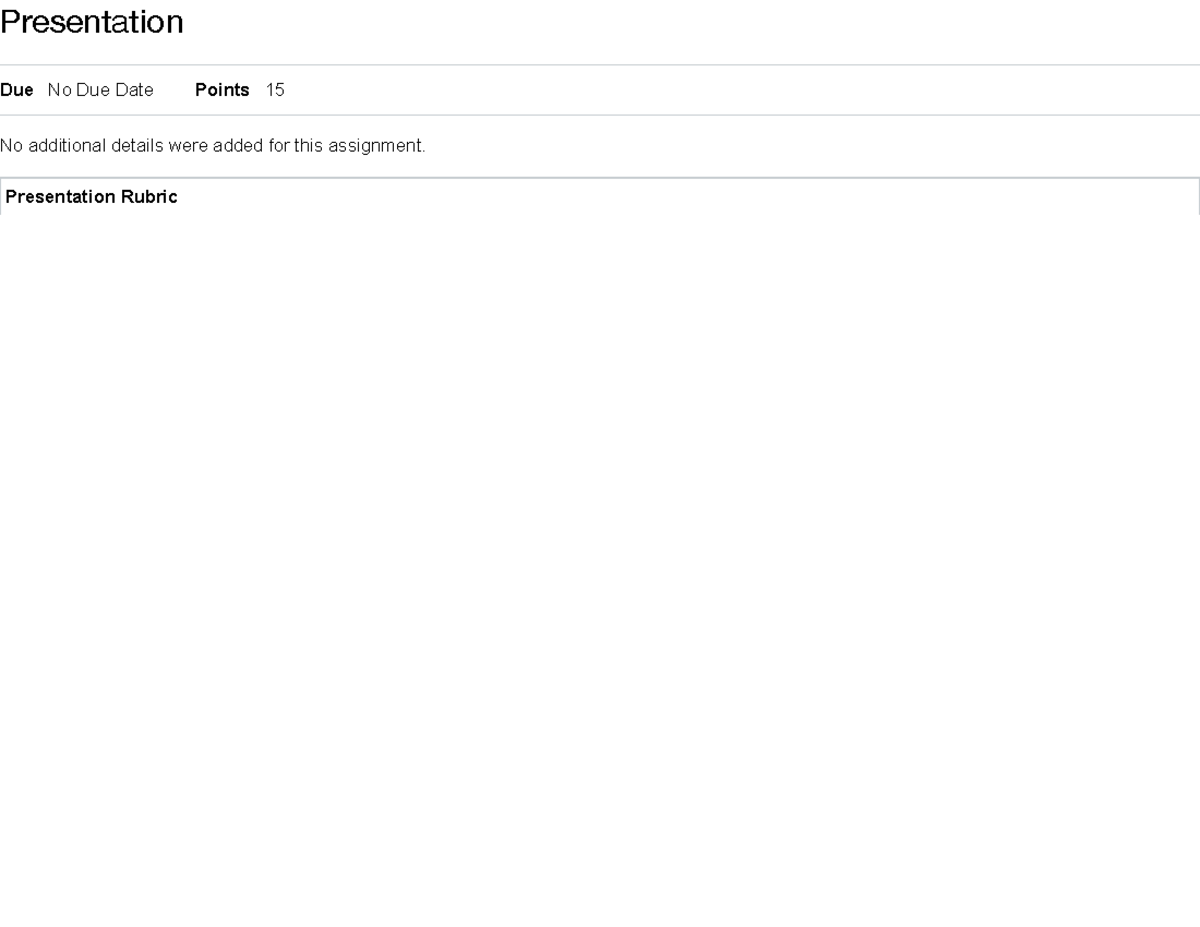The image is a screenshot of an assignment submission interface, presumably from an educational platform for managing school assignments. The background is predominantly white, creating a clean, minimalistic look. At the top left corner, the word "Presentation" is displayed in black, sans-serif font, followed by a light gray horizontal divider line. Directly below, bold text reads "Do," paired with "No due date" in a regular sans-serif font.

Another section underlines the "Points" value, which is indicated as "15" in non-bold text, with this segment also separated by a light gray horizontal line. Further down in smaller print, the statement "No additional details were added for this assignment" is visible, suggesting an incomplete or template format of the assignment. Another horizontal divider follows, beneath which "Presentation rubric" is written in bold text.

The overall impression is that the screenshot captures a partially filled-out template for submitting school assignments, indicating placeholders for information yet to be completed, such as due dates and additional task details.